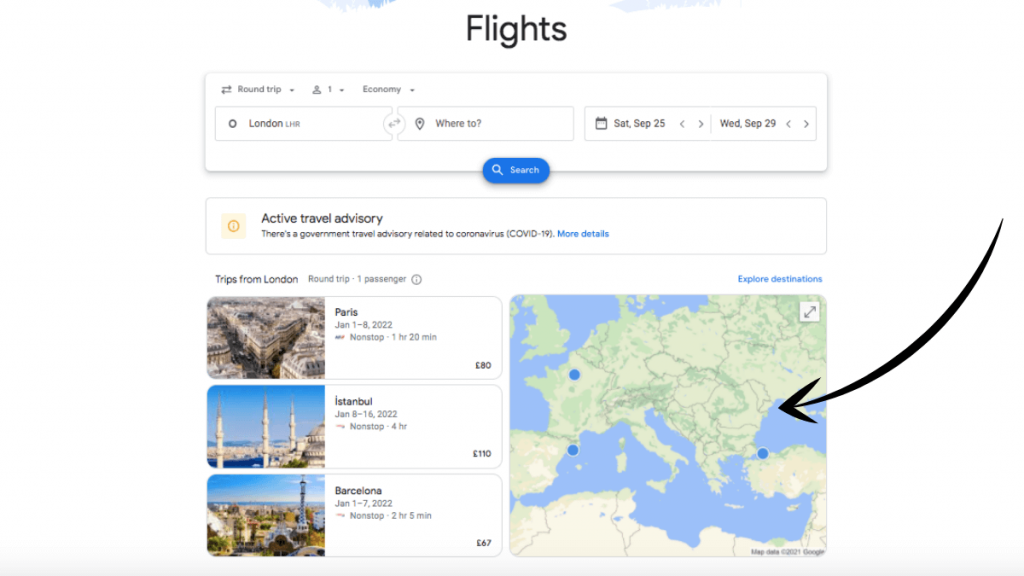The image showcases a detailed map characterized by varied hues of green, blue, and hints of brown. At its centerpiece is a dense area of high-saturation green, symbolizing a blend of land and thriving vegetation. This verdant expanse is encircled by blue regions, indicating water bodies that frame the terrain. Scattered across the map are three distinctive blue dots. At the top of the map, headers denote "Flights" and "Active Travel Advisory," guiding viewers on travel-related information. In the top right corner, a small icon signals the option to maximize the image, with a similar icon positioned at the bottom, offering the same functionality.